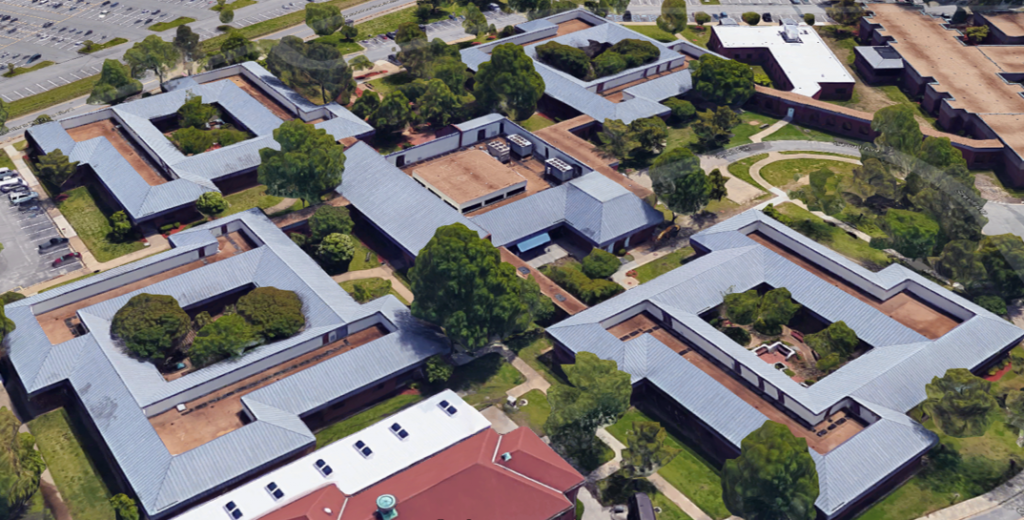An overhead photograph, likely taken by a drone, shows a complex of predominantly square-shaped, one-story buildings with both gray and light blue roofs. These buildings form a kind of grid pattern, with each having a hollow center resembling a courtyard. Within these courtyards, there's a mix of green shrubbery, trees, light brick plazas, and concrete pathways, some decorated with benches. Notably, one building at the bottom has a red roof featuring an array of skylights and a white portion. To the upper left of the image, a large parking lot is visible, with several empty spots and a few parked cars, including a white car, a blue car, and a black car. The entire scene is surrounded by well-maintained green lawns and additional trees between the buildings, contributing to a serene, organized appearance.